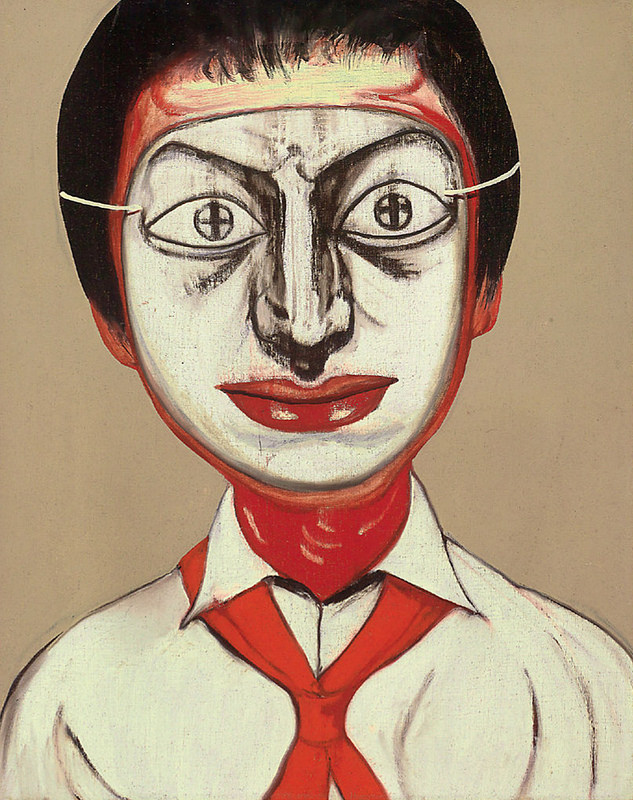A detailed portrait-style painting features a human figure, possibly a man, with short black hair and frayed strands near the ears. The background is a tan, dark sand color. The subject is seen from the chest up, dressed in a white collared shirt and a red necktie. The figure wears a disconcerting white mask held by visible strings. The mask has exaggerated, bug-like eyes with plus-sign pupils, forming a startled gaze, dark circles beneath the eyes, and a long, dark nose. The mouth is wide and painted bright red like lipstick, enhancing the overall unsettling appearance, reminiscent of a slightly eerie cartoon character.